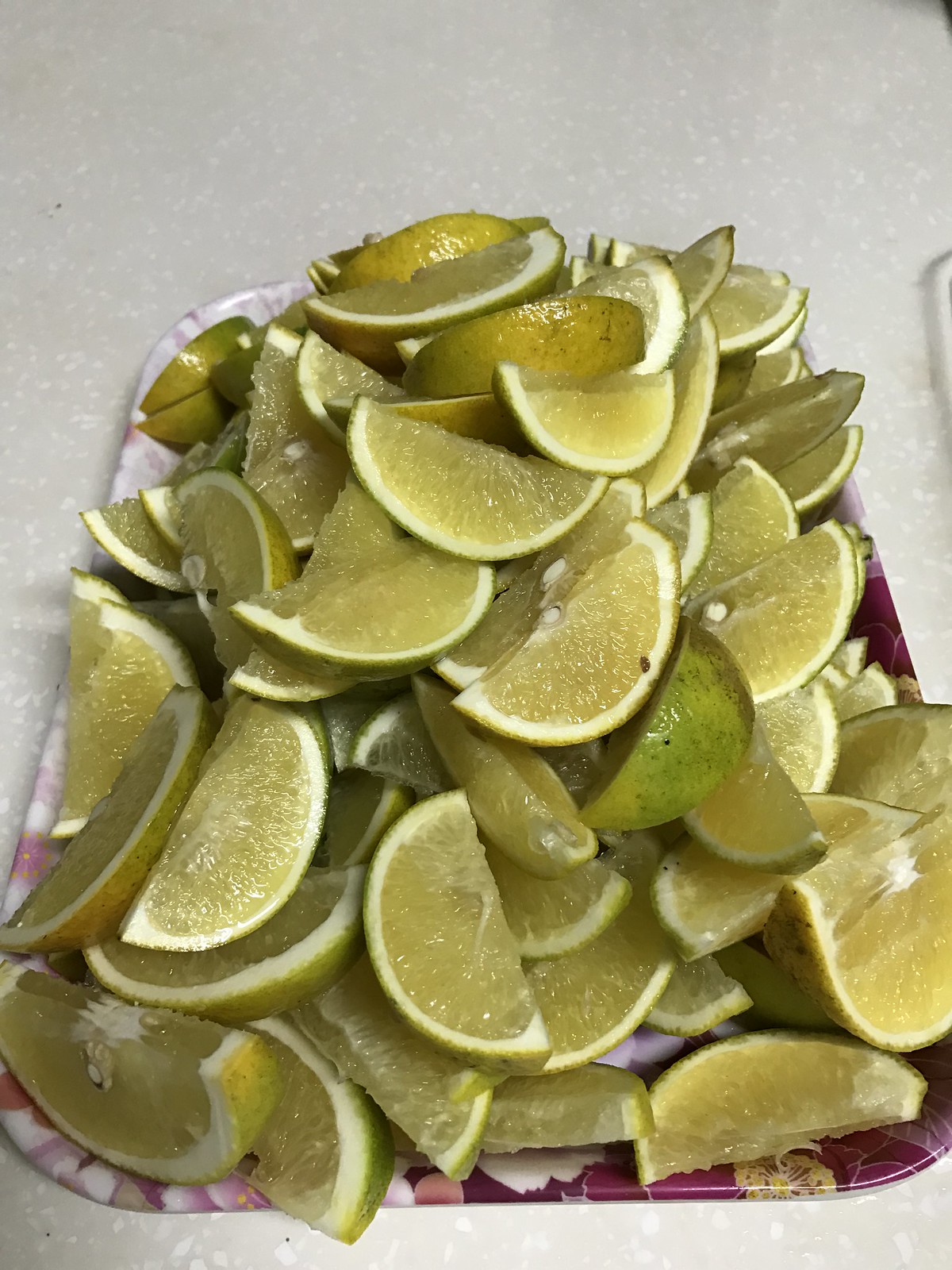This photograph prominently features a large pile of lime wedges, meticulously sliced into uniform sizes. The lime wedges, displaying their bright lime green rinds and dull yellowish-green, almost translucent flesh, are stacked high on a rectangular plate. The plate showcases a detailed and colorful floral design, incorporating shades of red, pink, and white. The limes are positioned with their rinds down and the juicy sections pointing upwards, some revealing small white seeds. The variety in the ripeness of the limes adds a subtle range of hues, from lime green to a light yellow with occasional brown specks. All this sits on an off-white countertop with small white dots scattered across its surface, providing a neutral backdrop to the vibrant display of citrus.